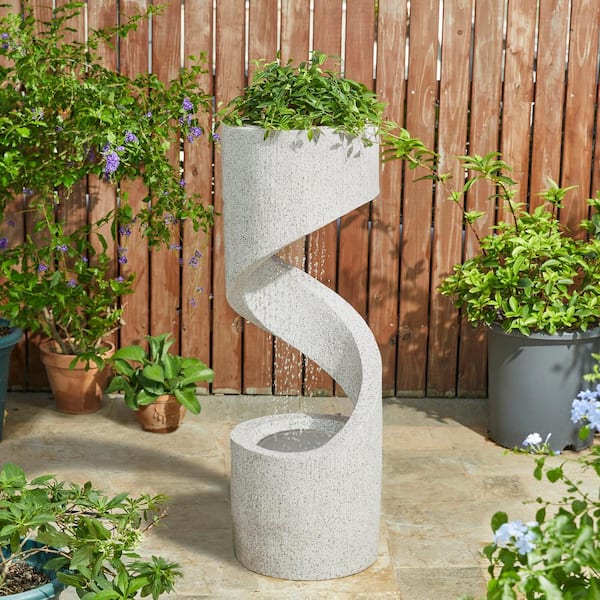In this outdoor photograph set in a yard, there's a prominent planter that functions both as a sculpture and a water fountain. The planter is light gray and swirled in design, starting from a base and spiraling upwards to a top container where vibrant green leaves grow. Water cascades down from the top, creating a waterfall effect into the base. Behind this feature, a wooden fence with slats allows light to filter through. Surrounding the main planter are several other pots, including a dark gray one, two rust-colored terracotta pots, and a blue one. These additional pots also contain lush green plants, with the terracotta ones displaying light purple flowers. In the foreground, there's a greenish-blue pot with a plant, contributing to the lushly green-scened area framed by the rustic fence.